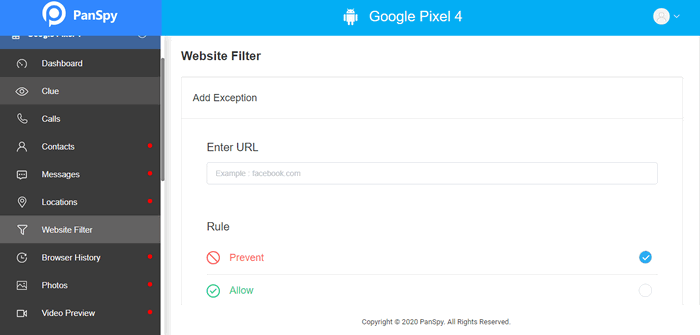This is a detailed screenshot of an interface showcasing two distinct sections: 
1. **PanSpy**: This section is indicated by a sidebar on the left with a logo and title. The sidebar has a dark gray background and includes a list of clickable options such as Dashboard, Clue, Calls, Contacts, Messages, Locations, Website Filter, Browser History, Photos, and Video Preview. The ‘Clue’ and ‘Website Filter’ options are highlighted in light gray. Items like Contacts, Messages, Locations, Browser History, Photos, and Video Preview have red notification dots next to them.
   
2. **Google Pixel 4**: This section takes up the main content area on the right side of the screen, set against an aqua blue background with a small robot logo. Below the header "Google Pixel 4" is a subheading titled "Website Filter," followed by an area labeled "Ad Exception" and an entry bar to input URLs. Additionally, the section contains a "Rule" heading with two radio buttons labeled "Prevent" and "Allow." The "Prevent" option is selected.